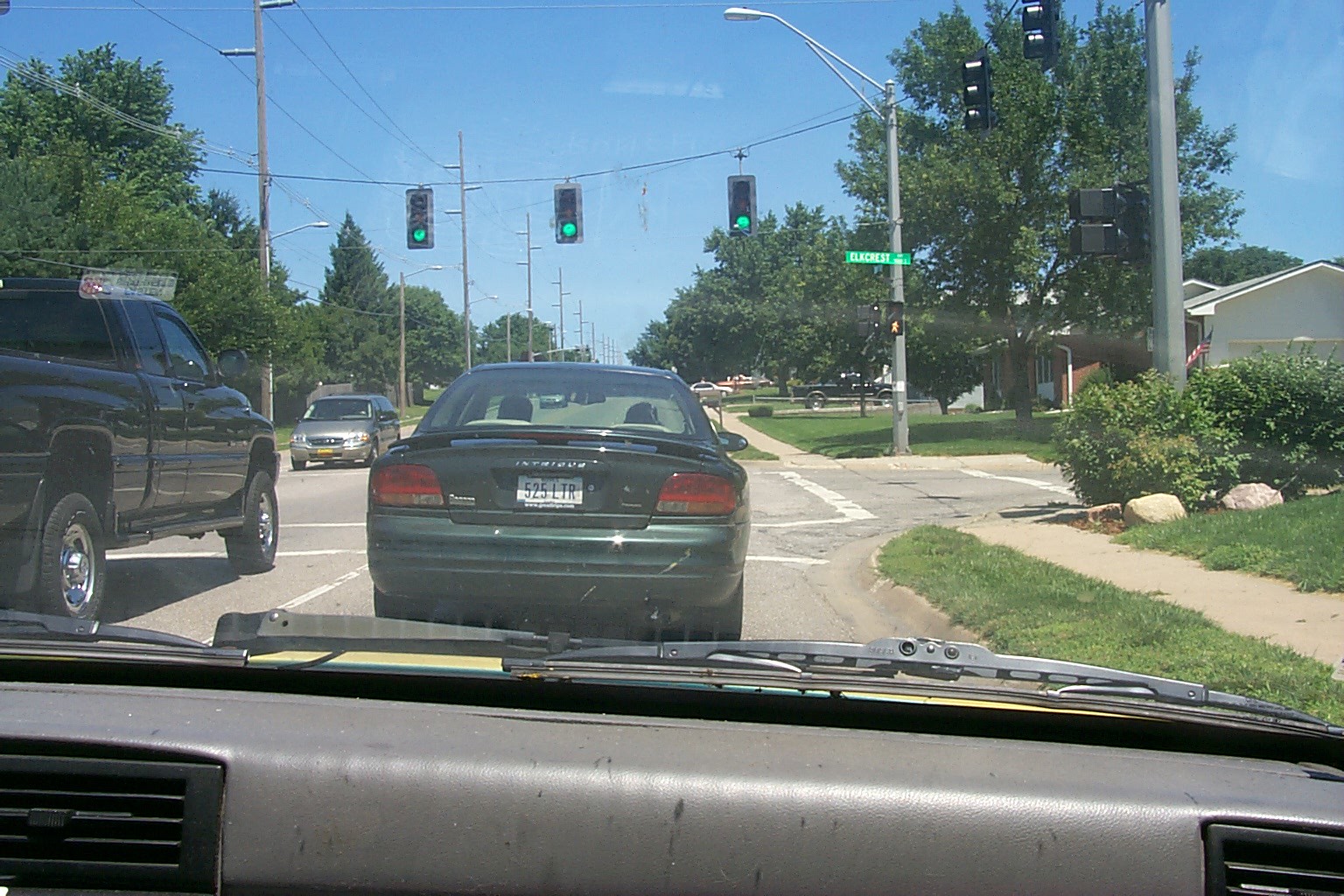This photograph, taken from inside a vehicle, captures a bustling street scene. The interior features a gray and black dashboard, framing a vibrant tableau outside the windshield. Directly ahead, a forest green car occupies the lane, flanked by a black pickup truck. Across the adjacent road, a goldish minivan is also visible. Overhead, a green stoplight hangs against a brilliant blue sky. The background showcases an array of power lines and houses, including a white one and another brick house adorned with white details. A "Walk/Don't Walk" sign is clearly displayed, along with a green and white street sign. Verdant elements like green grass, bushes, and trees add to the scene’s natural beauty. Additionally, white road markings are visible, enhancing the detailed depiction of this everyday moment.